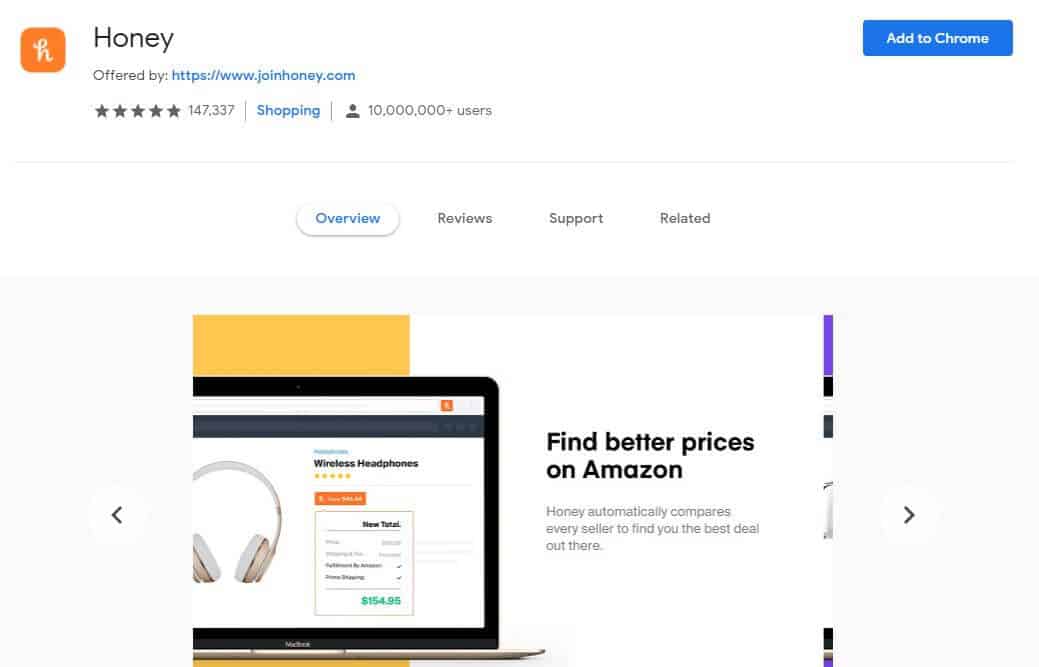This is a screenshot from the homepage of the Honey website, presented on a clean, white background. In the top left corner is an orange square featuring a white 'H' styled in a cursive-like lowercase font. To the right of this square, "Honey" is prominently displayed in large black lettering. In the top right corner, a blue tab with white text reads, "Add to Chrome."

On the left, beneath the Honey logo, "Offered By" is written in small black lettering, followed by a clickable blue link directing to https://www.joinhoney.com. Directly below this, the display includes five black stars and a user count of "147,337" next to a blue label marked "Shopping." It also mentions that the service has over "10 million+ users," accompanied by a profile icon.

Lower in the design, a horizontal menu is structured with options, starting from a white tab with blue text saying "Overview." Adjacent to it are tabs labeled "Reviews," "Support," and "Related" in black.

Towards the bottom left of the screenshot, an orange rectangular outline encloses part of the content, framing the image of a laptop screen. The laptop has a black border and a white top border, displaying a visual of white headphones on a blue background. To the right of the headphones, bold text reads "Wireless Headphones." Further to the right, central bold black text states, "Find Better Prices on Amazon." Below this, smaller black text explains, "Honey automatically compares every seller to find the best deal out there."

Additionally, small arrows on the left and right margins of the content allow for navigation, enabling users to scroll through images.